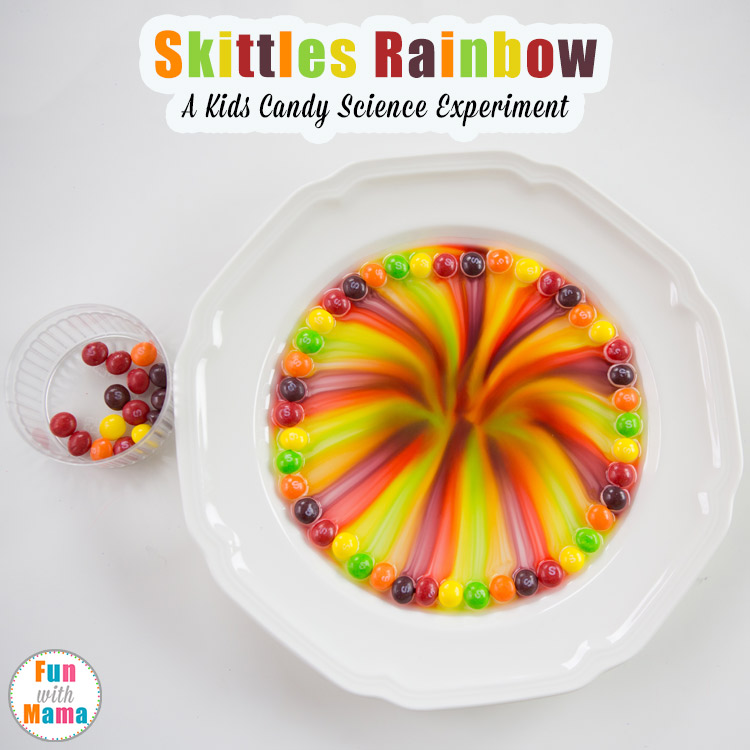The image is titled "Skittles Rainbow," highlighted in vibrant rainbow colors at the top, with "A Kid's Candy Science Experiment" written underneath in black. At the bottom left corner, a circular text reads "Fun with Mama." The central focus of the photo is a white plate positioned on a white table, the plate having a slightly dipped center filled with water. Surrounding the outer edge of the plate, different colored Skittles are neatly arranged, and as they dissolve, their colors bleed inward, creating a mesmerizing pattern reminiscent of a colorful vortex. To the left of the plate, there's a clear glass dish filled with additional untouched Skittles, suggesting they were not needed for the experiment.